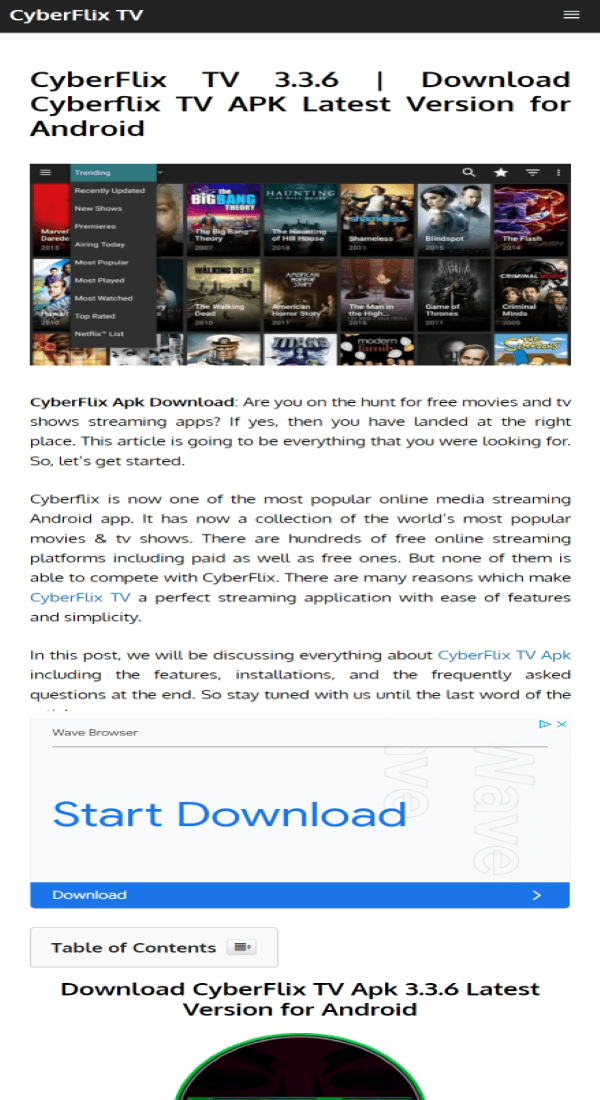This image is a mobile screenshot displaying the homepage of CyberFlix TV. At the very top, a thin black banner is visible with "CyberFlix TV" written in white font on the upper left corner. The main section has a white background featuring a title that reads, "CyberFlix TV 3.3.6 Download CyberFlix TV APK Latest Version for Android." Beneath the title, there is a screenshot showcasing a grid of available games. To the left of this image, a drop-down menu is visible.

Below this section, there are three paragraphs of text. The first paragraph starts with "CyberFlix APK Download" and asks, "Are you on the hunt for free movies and TV shows streaming apps?" The second paragraph notes that "CyberFlix is now one of the most popular online media streaming Android apps." The third paragraph indicates, "In this post, we will be discussing everything about CyberFlix TV APK including the features, installations, and frequently asked questions at the end."

Further down, a pop-up box appears with "Wave Browser" written at the top and "Start Download" in bold blue text, accompanied by a thin blue download button below it. Additionally, there's a "Table of Contents" button. At the bottom of the image, there is a half-circle icon outlined in green with a black center, displaying the text "Download CyberFlix TV APK 3.3.6 Latest Version for Android."